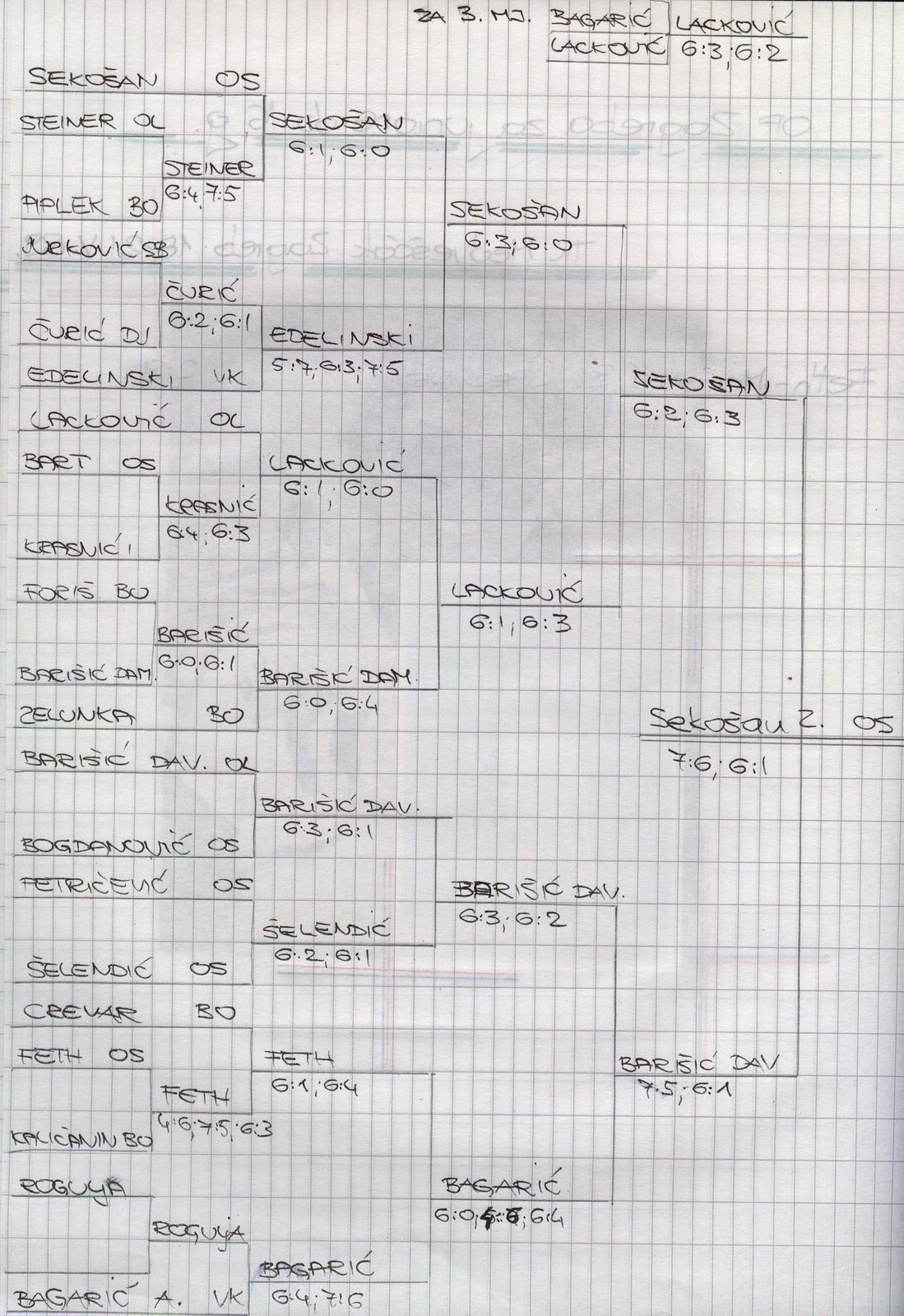This image appears to be a detailed tournament bracket chart drawn on legal-sized graph paper, with handwritten text in black ink. The graph paper has small, blue grid lines forming slightly elongated squares. At the top-left corner, the chart begins with names such as "Sikosin OS" and "Steiner," progressing through a series of interconnected brackets. The names "Overik" and "Piplik" appear in subsequent brackets, along with several other names that are difficult to read, possibly due to being written in a different language or script. The upper right of the paper includes more illegible text, potentially denoting betting odds or additional information, with a specific sequence noted as "6362." The chart starts with many names on the left, consolidating through several tiers toward the right, ultimately narrowing down to a final name, indicating the winner. Overall, the structure suggests a sports tournament or competitive event, tracking the progression of participants through successive rounds.